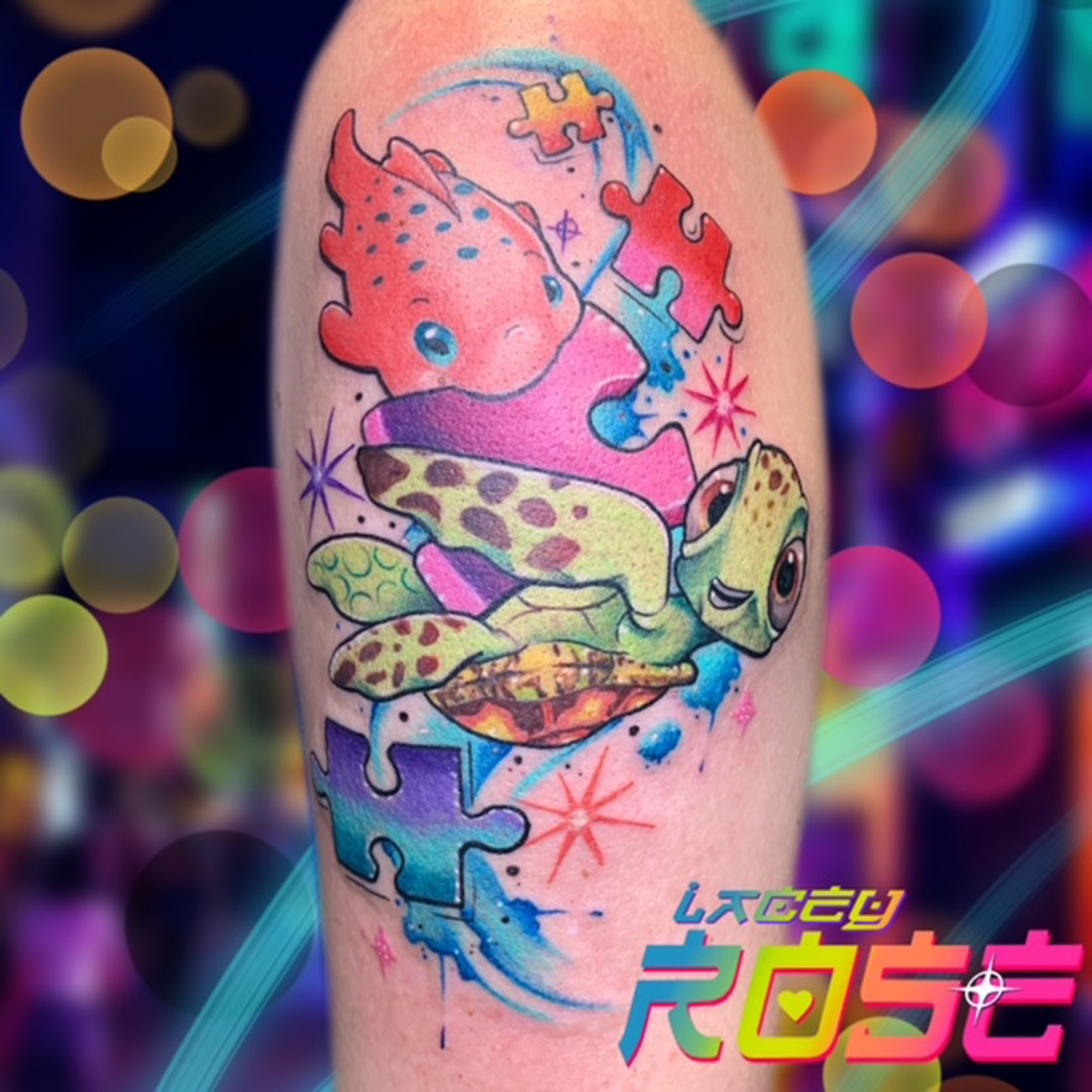This photograph captures a vibrant and intricate tattoo on what seems to be a section of a Caucasian person's limb, possibly the shoulder or bicep. The tattoo, rendered in new school art style, features a dynamic blue swirl that snakes downwards in a reverse S-shape, adorned with several puzzle pieces of varying colors. The top puzzle piece is yellow and orange, followed by a red and pink piece, and a large three-dimensional pink and purple piece. The final piece is purple and teal.

A small, cartoonish orange fish with blue spots and large blue eyes bites onto the pink and purple puzzle piece. Below, a baby sea turtle, resembling Squirt from Disney Pixar's "Finding Nemo," smiles broadly as it holds the puzzle piece with its fins. The turtle is depicted with vivid green shading and expressive eyes.

Encircling these main elements are waves of blue water and starbursts in purple, orange, and pink. A notable detail is the name "Lacy Rose" written in a gradient of blue, green, yellow, orange, and pink in the lower right corner of the tattoo. The background of the image features glossy, shimmering lights and a bokeh effect with circles in various colors, including bright yellow, gold, pink, and blue, set against a dark blue backdrop.